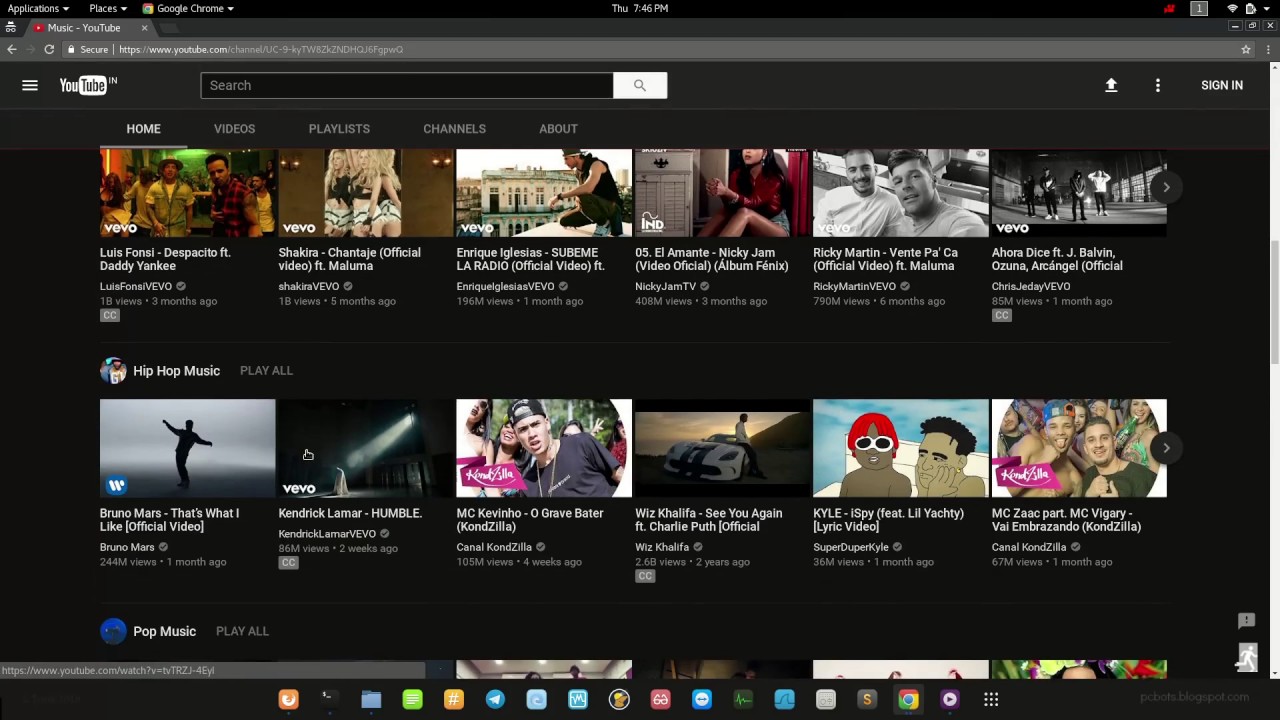Here is the cleaned-up and more detailed caption:

The image is a horizontally rectangular screenshot of a website taken in dark mode, featuring a black background. In the top left corner, there is a drop-down menu labeled "Applications," followed by another drop-down menu labeled "Flexes," and then "Google Chrome," each accessible via their respective drop-downs. At the center top of the frame, the time "Thursday 7:46 p.m." is displayed. 

Below the time, there is a single browser tab titled "Music YouTube" situated on the left side. Directly beneath the tab, the website address bar is visible, further emphasizing the dark mode aesthetic.

The main content of the screenshot is the YouTube Music interface. At the top, there is a search field specific to YouTube Music. Below this search bar, there are two rows containing six different options each. The options on the first row do not have a heading, while the second row is labeled with the heading "Hip-hop Music." 

Just above these rows, navigation options are available, labeled "Home," "Videos," "Playlists," "Channels," and "About," allowing users to explore different sections of the YouTube Music channel.